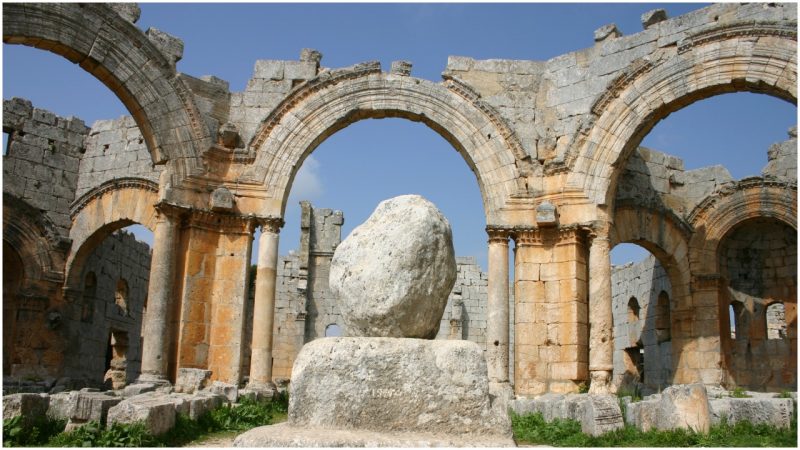The photograph captures a vibrant, sunlit scene of ancient ruins, showcasing an intricate collection of stone arches and pillars, some of which exhibit an orangish patina, especially near their bases, transitioning to gray higher up. Central to the image stands a striking large white rock with a potato-like shape perched atop a square white pedestal marked with a partially legible date starting with "19." Surrounding the pedestal is a patch of green grass that contrasts with the stone structures. The background reveals additional incomplete walls of gray stone blocks, reinforcing the sense of historical decay. The bright blue sky and a tiny cloud add to the vividness of the scene, highlighting the beauty and antiquity of what might have once been a grand temple or bathhouse, now in picturesque ruins.